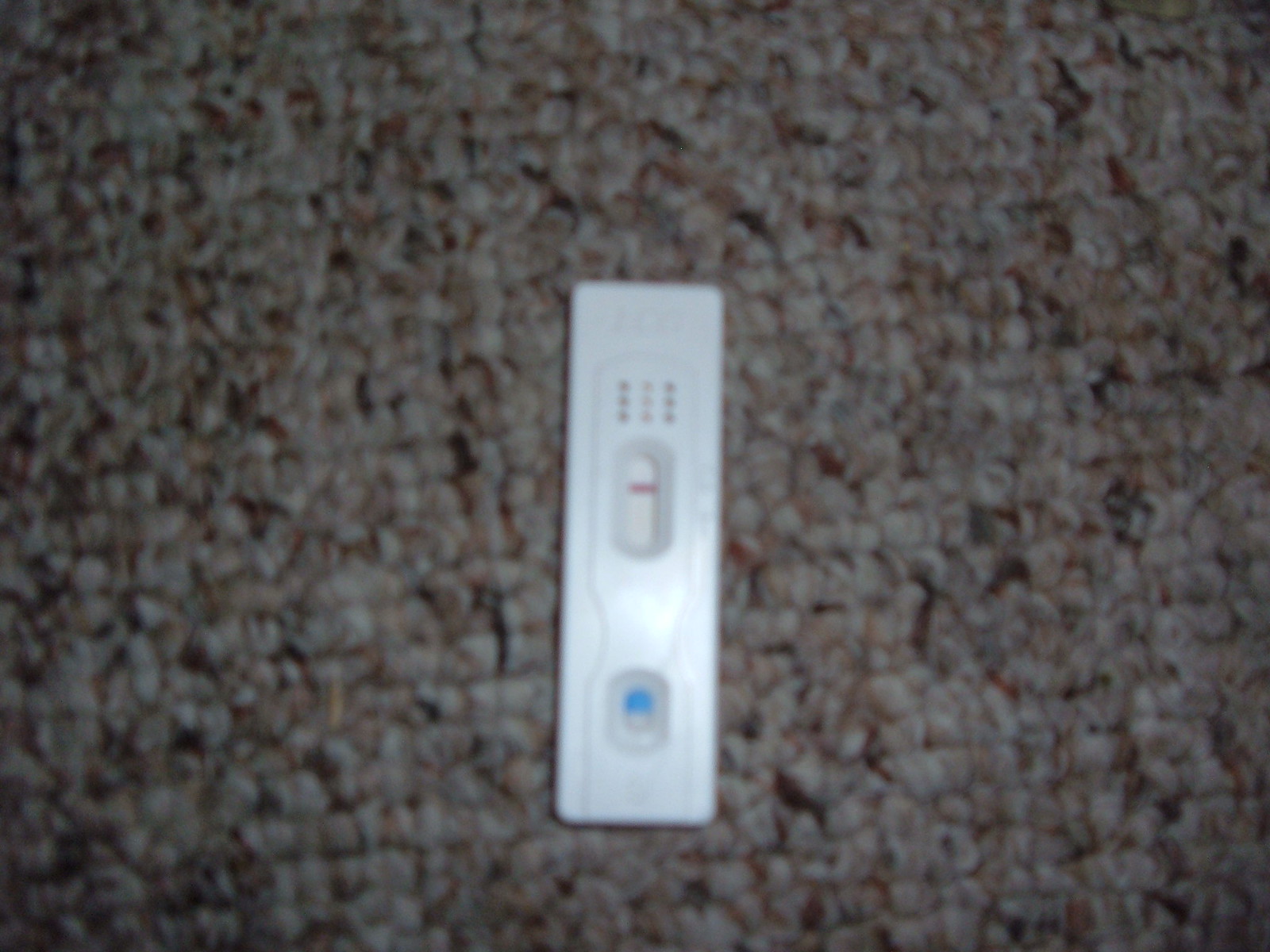The image captures a slightly blurry view of what appears to be a test device, possibly a home COVID test, placed on a textured surface. The surface resembles a light beige to dark brown patterned carpet or upholstered mat with a mixed, uneven texture. At the center of the image is a rectangular, white test apparatus featuring two distinct windows.

The upper window is an elongated, rounded rectangle - almost oval in shape - etched with subtle branding or instructions above it. Below this, three columns of three dots each are positioned just above the upper window, possibly serving as markers or indicators.

The top window features a background off-white tint with a singular red line running horizontally across it, likely functioning as a control line. Further down, there is a second, smaller, oval-shaped window. This secondary window displays a semi-blue, semi-white background, typical of areas where users deposit a sample, reminiscent of common home tests. The blue indicates where the drops were placed, while the upper section of the panel appears to be where the result would typically manifest.

In the current state of the test shown, only one red control line is visible, with no additional lines to indicate a positive test result.